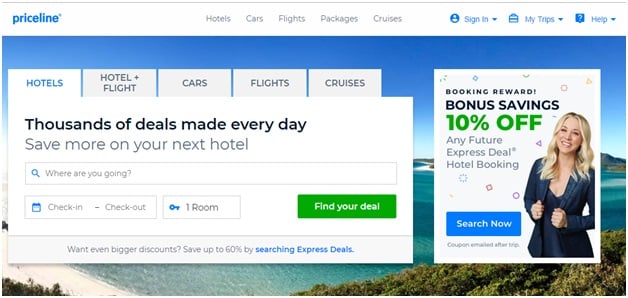The image displays the homepage of the Priceline website. Dominating the top left corner, the Priceline logo is prominently displayed in blue text. Adjacent to the logo are five navigation categories listed in gray text: Hotels, Cars, Flights, Packages, and Cruises. To the far right of this navigation bar, there are three user options in blue text: Sign In, My Trips, and Help.

Directly below this navigation bar, there are additional categories listed: Hotels, Hotel + Flight, Cars, Flights, and Cruises. Beneath this, within a white rectangular banner, is the message in gray text, "Thousands of deals made every day - Save more on your next hotel."

Further down, a prominent search bar asks "Where are you going?" This section includes a check-in and check-out date filter. To the right of the date filters is a blue key icon with text indicating the number of rooms, set to "one room" by default. There is a green rectangular button labeled "Find Your Deal" that finalizes the search input.

To the right of these features, prominently displayed in a white square popup, is a "Booking Reward" offer, boasting "Bonus savings" with "10% off" any future Express Deal hotel booking, highlighted in green. Below this popup is a blue search button for additional navigation.

The overall background of the website is a picturesque scene featuring a tranquil body of water. A stretch of beachfront is visible along with an island in the distance, all beneath a clear blue sky, contributing to a serene and inviting ambiance.